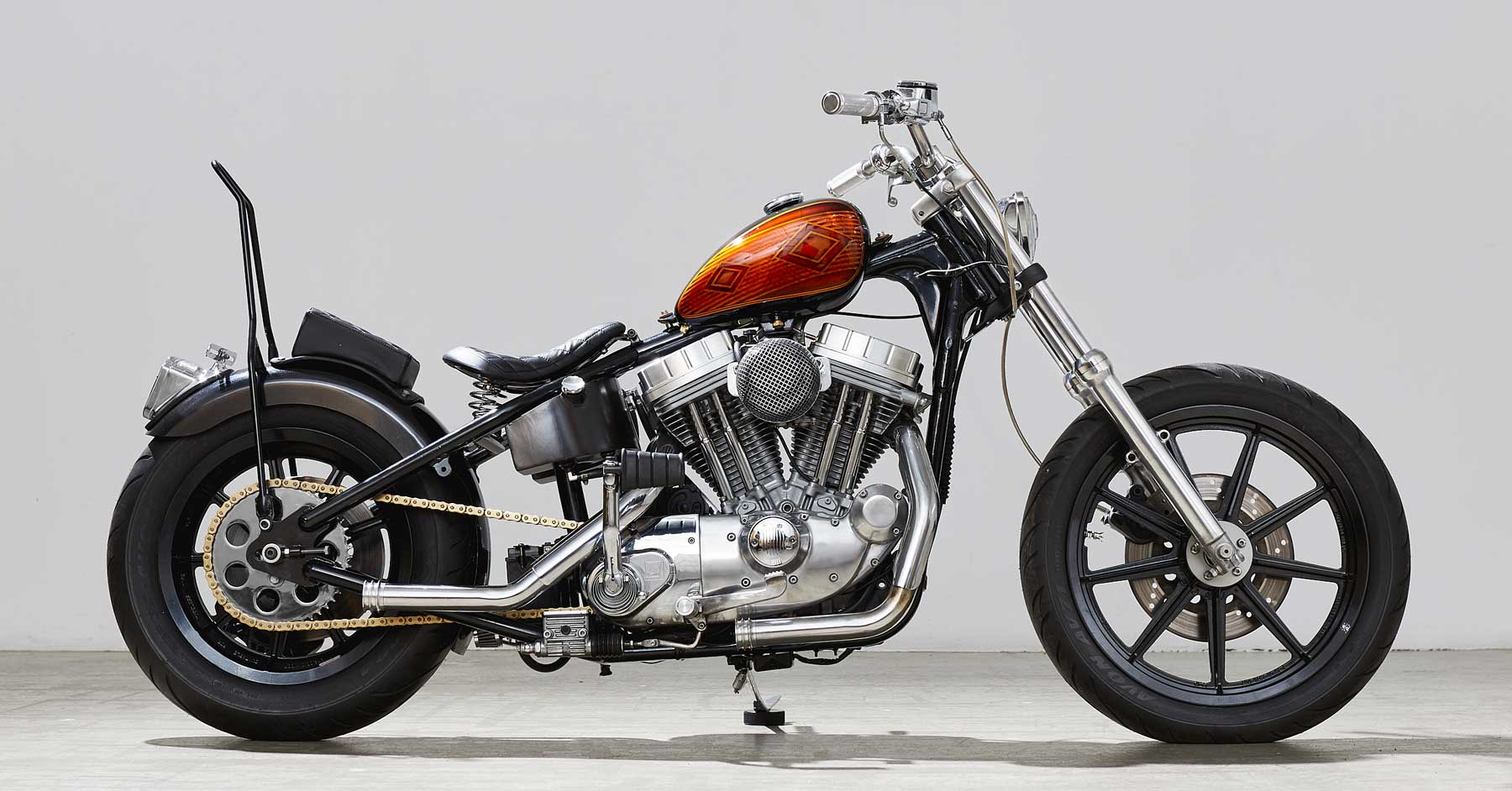The image features a detailed, photorealistic side view of a custom-built motorcycle set against a flat, light gray concrete ground and a plain white wall. The predominantly chrome motorcycle showcases a distinctively small gas tank, painted in an eye-catching orange marble pattern with two diamond shapes. The seat is black, positioned low and angled upward towards the tank. A large black bar extends from the rear wheel, serving as a potential backrest. The motorcycle, with its sleek design, includes additional features like big, flat, fat black wheels and a tail light. The overall composition highlights the contrast between the bike's gleaming chrome and the singular vibrant orange element, emphasizing its modern and striking aesthetic.